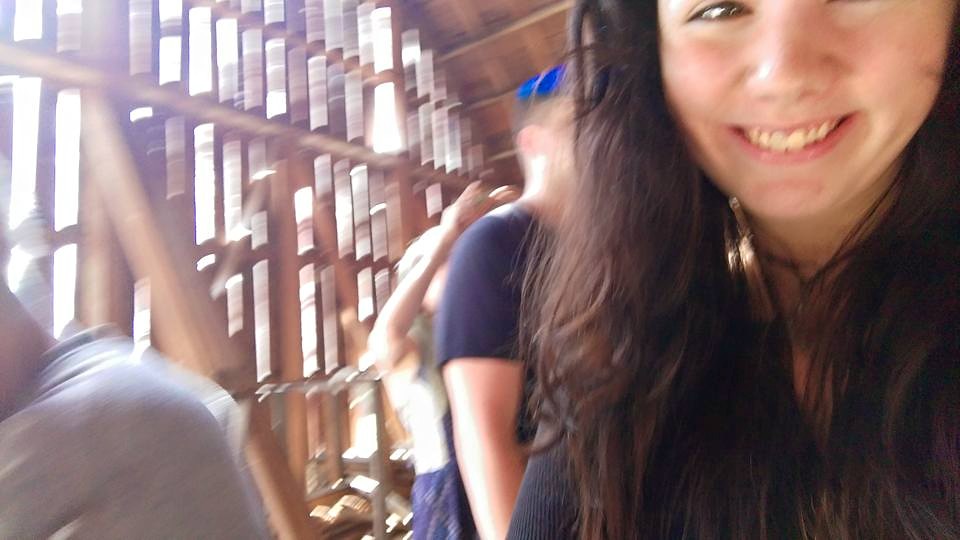The photograph captures a lively scene with people in motion. In the foreground, there is a close-up of a woman, occupying about a third of the frame, from eye level down. Her face, hair, clothing, and earrings are clearly visible, providing a focal point for the image. Behind her, slightly to the right, a man is in mid-movement, resulting in a blurred depiction. You can make out his ear, hair, part of his cap, and one t-shirted arm. Further back, a woman is partially obscured by the man, with only her raised arms visible, suggesting she might be dancing. On the left side, part of another man's shoulder blade and the back of his neck are visible. In the background, light filters through a lattice wall, adding a textured and illuminated backdrop to the bustling scene.